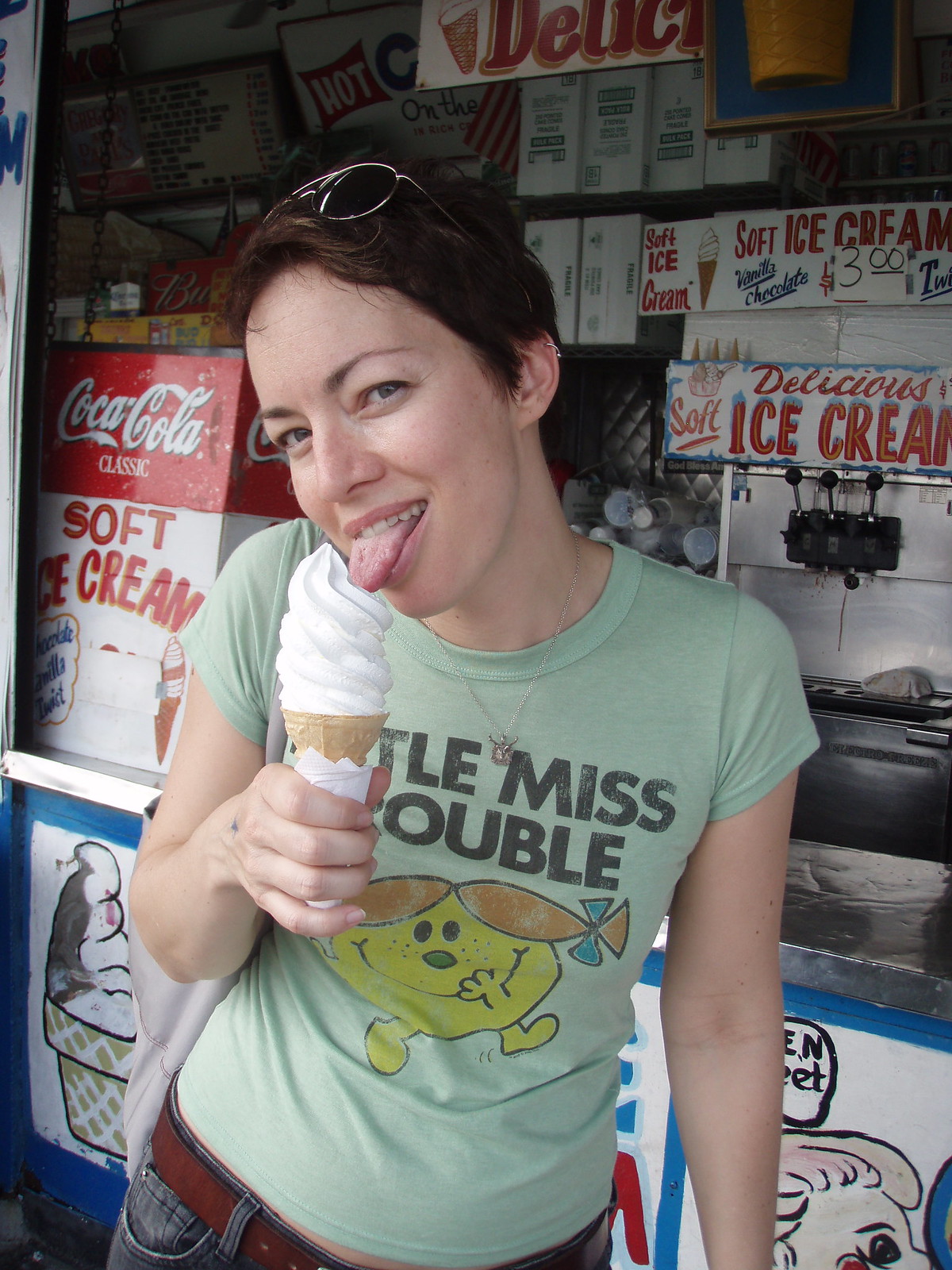This photograph captures a woman standing in front of an ice cream shop, wearing a light green t-shirt with text that reads "Little Miss Double" and a cartoon drawing on it. She is also dressed in blue jeans, with a gray bag slung over her shoulder. The woman, who has short hair, sports black sunglasses perched on her head. She is holding a soft-serve cone with a vanilla swirl in one hand and playfully sticking out her tongue as she takes a taste of the ice cream. In the background, several ice cream dispensing machines from the shop are visible, adding context to the joyous moment she is experiencing.